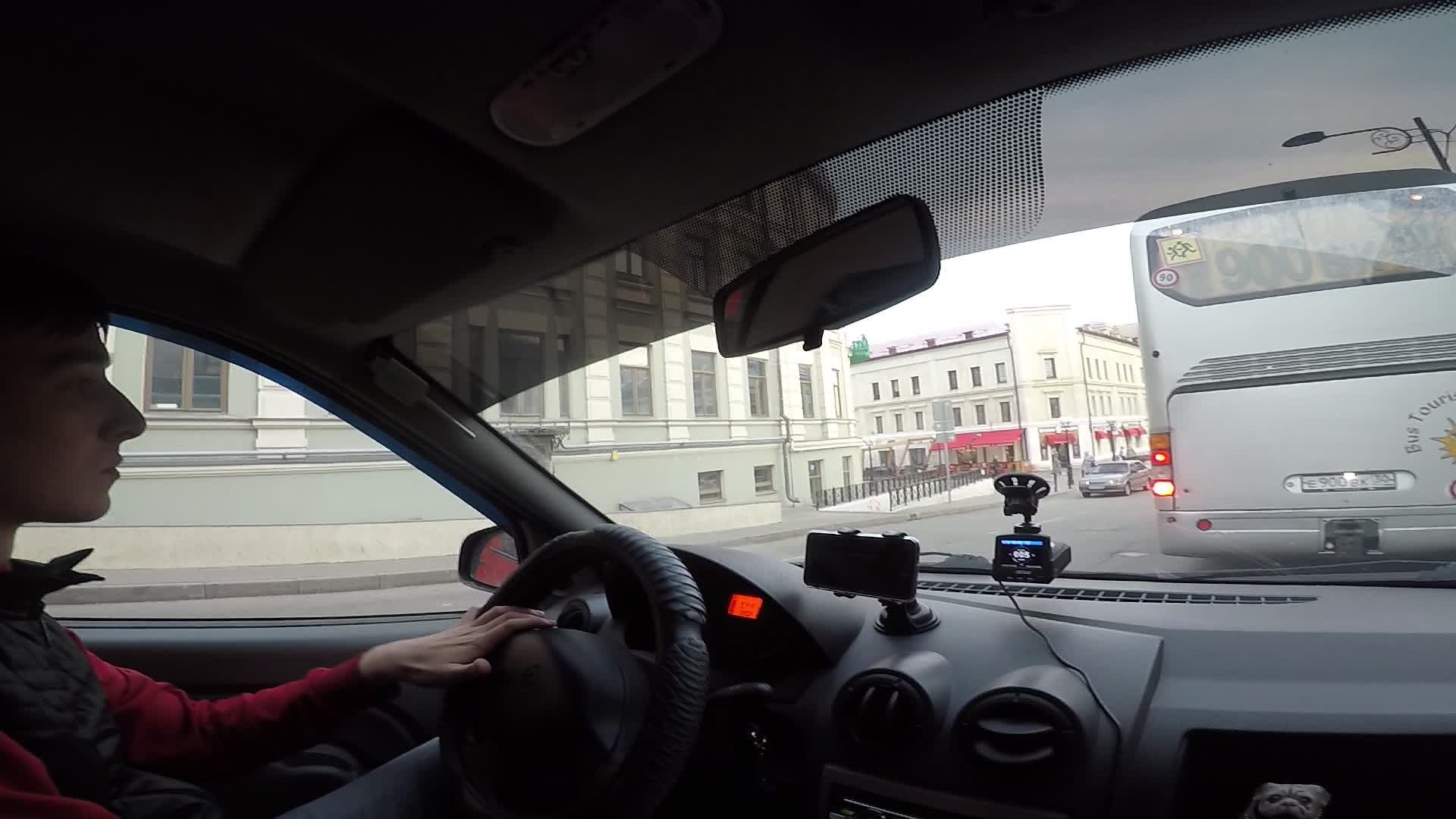The image captures a scene from the passenger's perspective in a vehicle. A Caucasian-looking male is seated in the driver's seat, wearing a long-sleeved burgundy-colored shirt underneath a black sleeveless zip-up vest. His left hand rests on the black steering wheel, which is covered with a steering wheel cover. He has light white skin, dark brown hair, and a slightly prominent nose, appearing in partial shadow. 

The interior of the vehicle is predominantly black and gray, with a digital display emitting an amber glow visible behind the wheel. A cell phone is secured in a holder attached to the dashboard, and another device, possibly a GPS or radar detector, is mounted with a suction cup to the center of the windshield, connected by a visible cord.

The scene outside shows an urban setting with the vehicle positioned behind a city bus that has gray bodywork and red taillights. To the left, large three-story apartment buildings are visible with red awnings and bike racks or other metal structures in front. The overcast sky is filled with off-white clouds, adding to the urban atmosphere.